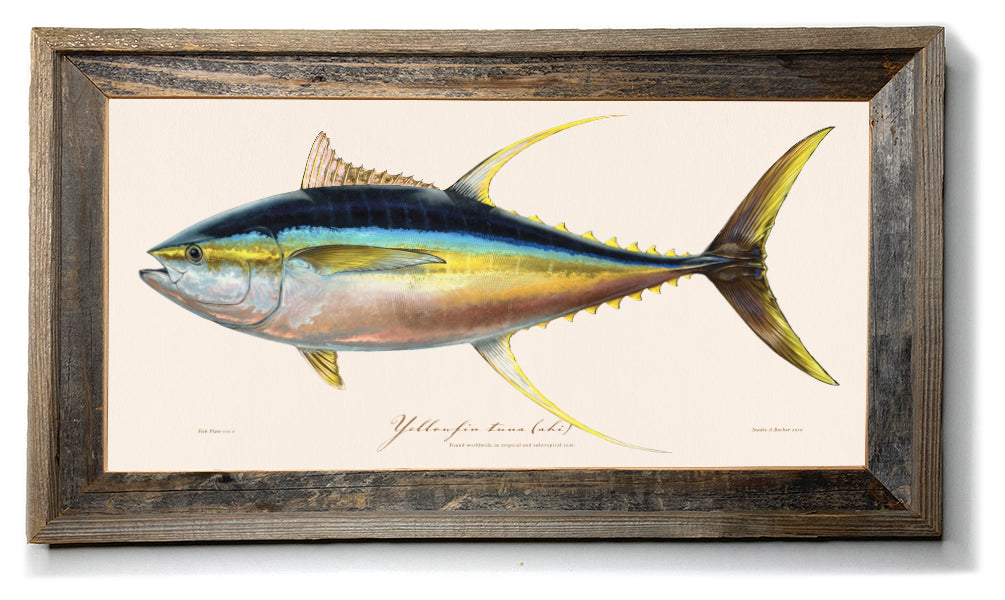This is a framed picture of a yellowfin tuna, depicted in a detailed and colorful painting or drawing. The fish faces left with its mouth open, showcasing its blue, silver, and gold hues, along with a distinctive yellow stripe running along its body. The fish's tail and fins all include shades of yellow, which is characteristic of a yellowfin tuna. Specifically, it has two sets of yellow fins—one in the middle and one towards the back of its body—along with a light blue stripe above the yellow and a darker bluish-gray top. The dorsal fin is notably up, and the fish’s eye on the left side is clearly visible. The background of the picture is white, and the image is encased in a darkish brown, rustic wooden frame, which appears fairly thick and possibly aged. Although there are labels below the fish and on the bottom left and right sides of the frame, they are unreadable in this image. Only the framed picture itself is visible, without any indication of its surrounding environment.